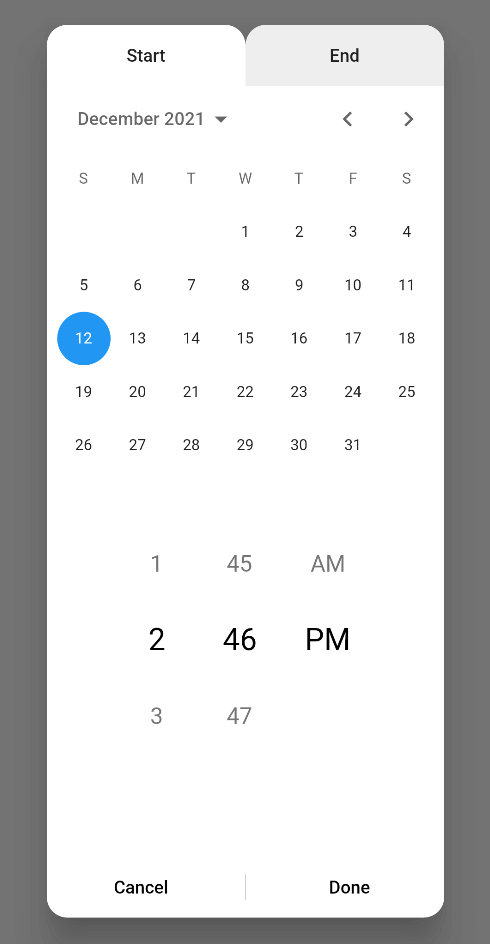This is a screenshot from a mobile device, oriented in portrait mode, with a medium grey background. At the top of the screen, there are two tabs: "Start" and "End." The "Start" tab is currently selected, displayed with a white background and black text. The "End" tab has a light grey background with black text.

This screenshot likely depicts a trip planning or appointment scheduling interface. The calendar is set to December 2021, with a blue circle highlighting the date December 12th. The number 12 appears in white within the blue circle, indicating it has been selected. The start time is specified as 2:46 PM, shown in large, black font, while other numbers on the screen are smaller and grey.

At the bottom of the screen are options to "Cancel" and "Done," both in black text, with a faint vertical line separating them. Additionally, near the top-right corner beside "December 2021," there is a drop-down menu for selecting the month and year, accompanied by left and right arrows for navigating between different months.